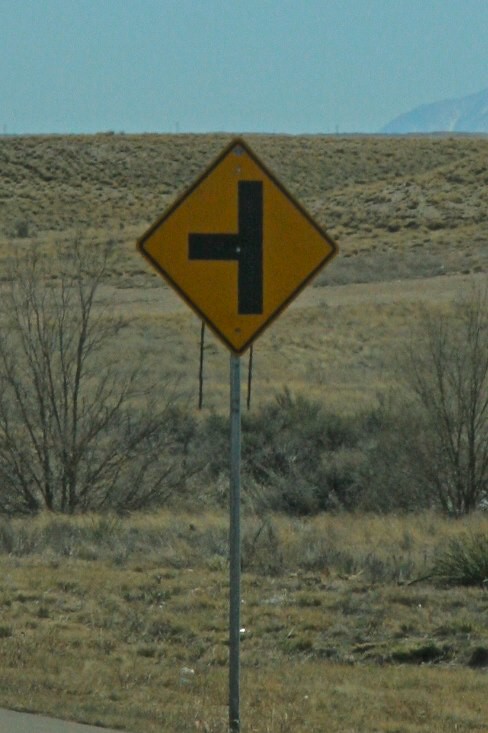This photograph features a yellow diamond-shaped traffic sign mounted on a slender steel pole by the side of a remote road. The sign depicts a black “T” shape tilted to the left, indicating an upcoming intersection where the road continues straight, but a left turn is possible. The setting behind the sign includes a field of beige and green hues, consisting of grass and shrubs, suggesting either a desolate or transitional landscape, with some sparse foliage. Beyond the immediate vegetation, grassy hills rise up, gradually leading to distant rolling mountains under a partially overcast, light blue sky. The entire scene suggests a quiet, isolated area, with the natural elements dominating the surroundings.